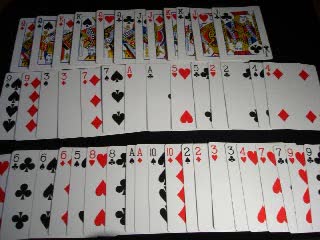The image depicts a meticulously arranged grid of standard playing cards laid face up on a black surface, likely a table. The cards are organized in three horizontal rows. 

In the topmost row, 12 cards extend almost to the right edge, leaving a small gap in the top-right corner. These cards, ordered from left to right, include: Queen of Diamonds, Queen of Spades, King of Diamonds, King of Spades, Queen of Hearts, Queen of Clubs, Jack of Spades, Jack of Diamonds, King of Hearts, King of Spades, Jack of Hearts, and Jack of Spades. 

The second row stretches entirely across the image, displaying: 9 of Spades, 9 of Diamonds, 3 of Spades, 3 of Diamonds, 7 of Diamonds, 7 of Spades, 8 of Hearts, 8 of Clubs, 5 of Hearts, 5 of Clubs, 2 of Hearts, 2 of Clubs, 4 of Clubs, and 4 of Diamonds.

The final, bottom row is similarly uninterrupted, but one card's value is obscured, showing only the suit of Hearts. The visible cards are: 6 of Clubs, 6 of Spades, 6 of Diamonds, 5 of Clubs, 8 of Hearts, 8 of Clubs, 8 of Spades, 8 of Diamonds, Ace of Diamonds, 10 of Spades, 10 of Diamonds, 2 of Spades, 2 of Diamonds, 3 of Hearts, 3 of Spades, 4 of Hearts, 7 of Hearts, 7 of Spades, 9 of Hearts, and 9 of Spades.